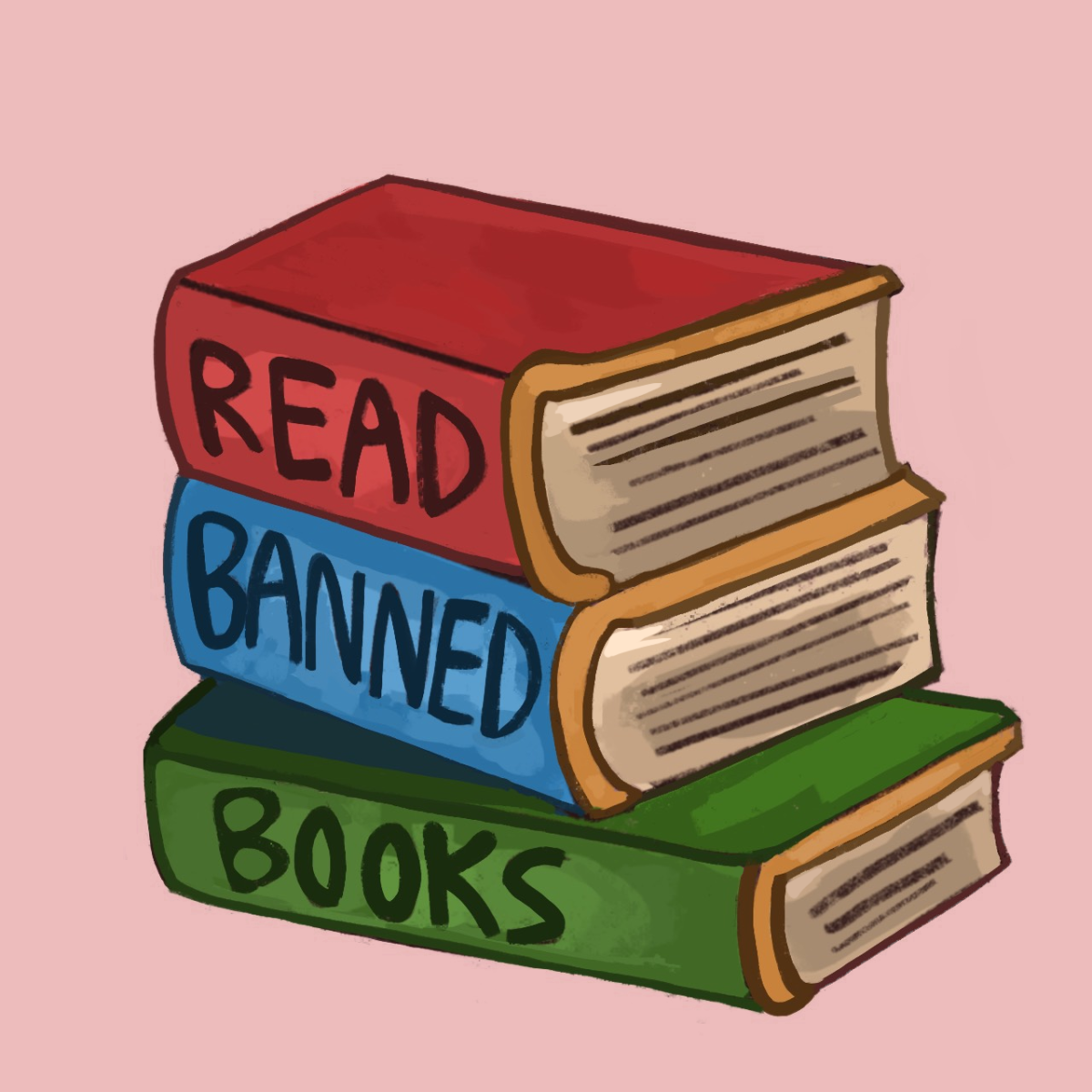The image features a simple yet striking illustration set against a dull pastel pink background. Central to the image are three cartoon-style books stacked one on top of the other, each adorned with vivid colors and detailed trims. The topmost book is red with gold trim and a brownish tint along its page edges, bearing the word "READ" in uppercase, prominent letters on its spine. Directly beneath it lies a slightly larger blue book, similarly trimmed in gold, with the word "BANNED" printed on its spine. The bottommost book is green and, while thinner yet broader than the others, completes the stack with the word "BOOKS" on its binding. Together, these books form the phrase "READ BANNED BOOKS," a clear and compelling message against censorship. The simplistic graphic design, featuring evenly spaced lines to mimic the pages in each book, enhances the visual impact of the call to action.